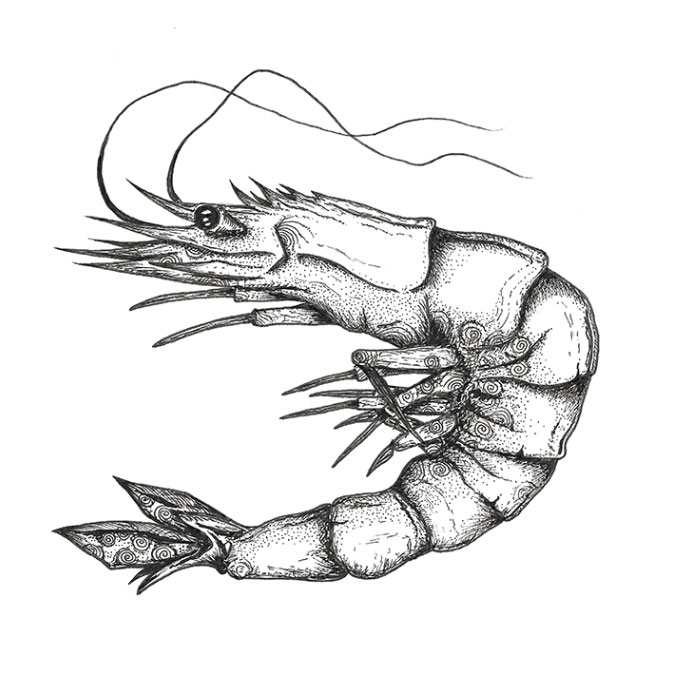This detailed black-and-white pencil drawing vividly depicts a shrimp-like sea creature from the side, curling gracefully from the upper left corner to the lower right. The creature is illustrated with exceptional detail, showcasing the segmented tail with distinctive circular markings—reminiscent of shrimp anatomy—leading up to the articulated exoskeleton divided into eight clearly-delineated sections. The central portion reveals numerous appendages and legs, precise in their arrangement, while the head features striking details like prominent eyes and intricate antennae that sweep back over the body. Additionally, the creature boasts delicate feelers and fine hairs near the head, enhancing its lifelike appearance. Though there's some ambiguity whether the creature is a shrimp or crawfish, the drawing's precision and skillful execution leave a lasting impression.